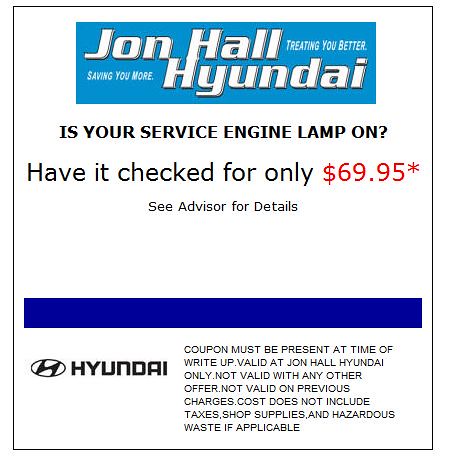This image is an advertisement for John Hall Hyundai featuring a promotional coupon offer. At the top of the ad, a light blue banner prominently displays "John Hall Hyundai" alongside the slogan "treating you better, saving you more" in blue text. Below this banner, in black text, it asks, "Is your service engine lamp on?" and offers a diagnostic check for only $69.95, with the price highlighted in red. Despite an asterisk next to the price, no additional explanation is provided. Directly underneath, it advises readers to "see advisor for details." A royal blue horizontal bar separates this section from the bottom of the ad, where the Hyundai logo and the word "Hyundai" are situated on the left. To the right, smaller text details the coupon conditions: "Coupon must be present at time of write-up, valid at John Hall Hyundai only, not valid with any other offer, not valid on previous charges, cost does not include taxes, shop supplies, and hazardous waste if applicable."